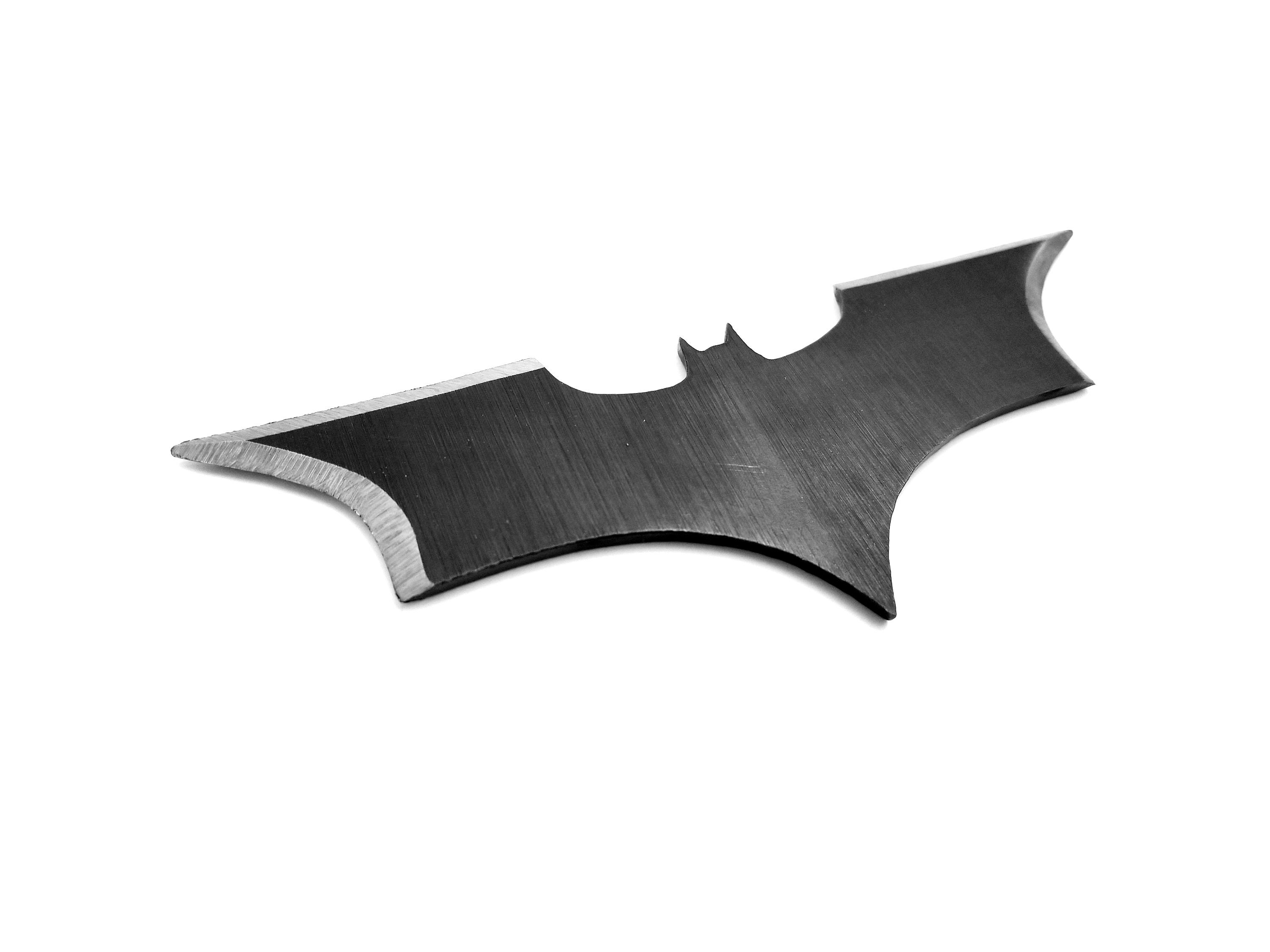A meticulously detailed image showcases a cutout of a black bat, reminiscent of the iconic Batman logo. This bat, possibly fashioned from wood or metal, features outstretched wings with sharp, light gray beveled edges. The texture reveals fine striations across the bat's body, suggesting a carefully crafted material. Its distinctly round head, adorned with two small ears, points northwards while its pointed tail aims south. Significant details include a slight scratch on the left side of its body, enhancing its realistic portrayal. The absence of a background and a faint shadow beneath the bat emphasize its form, creating a striking, minimalist visual.